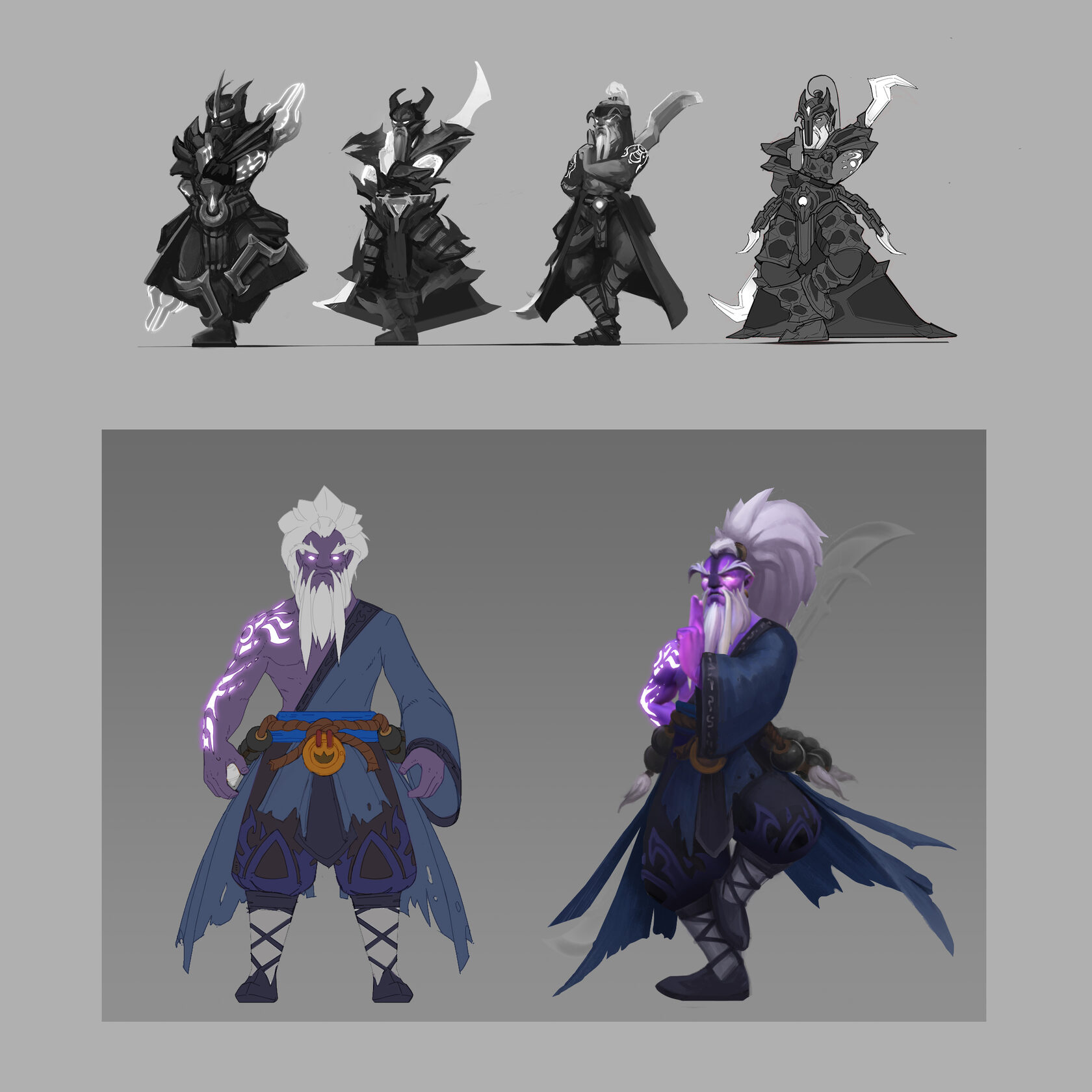This is a detailed computer-generated character design poster featuring six individual figures. The upper section showcases four 3D and 2D grayscale models, each of them in various martial arts poses, adorned with different variations of Japanese-style armor and cloaks. The characters hold distinct weapons, and the intricate designs highlight their detailed armaments and flowing attire.

In the lower section, two fully rendered characters are depicted in color. Both characters, old men with glowing white eyes, boast striking features including large heads of long grey hair tied into ponytails, and prominent, flowing white beards. Each has intricate, luminous tattoos running down their arms. The character on the left, who has purple skin and an ancient martial artist’s demeanor, is dressed in blue monk robes and stands in a martial arts pose, wielding a weapon. He also wears a distinctive white circular object suspended from a rope belt. The overall aesthetics combine elements of ancient Chinese and Asian cultures, indicating a fantasy setting, likely for a video game.